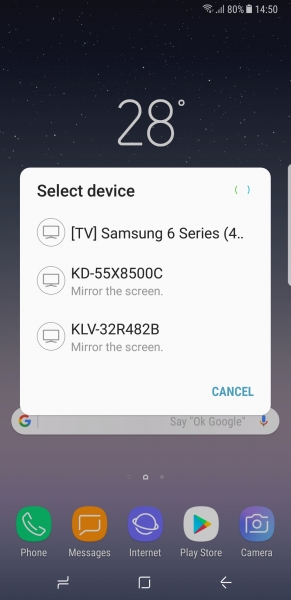The image depicts a smartphone screen displaying various elements and options. At the top of the screen, there are Wi-Fi signal bars, phone signal strength indicators, an 80% battery level icon, and the time displayed as 14:50 (2:50 PM). The weather is shown, indicating a temperature of 28 degrees.

Below this information, there's a pop-up menu labeled "Select Device" for screen mirroring options. The devices listed for mirroring include:
1. A Samsung 6 series TV.
2. A KD model TV (KD 556 55X 8500).
3. Another KD model TV (KLV 32R4A2B).

Each listed device has a TV icon next to it. At the bottom of the pop-up menu, there is a "Cancel" button highlighted in blue.

Further down, there's the Google search bar, followed by a row of app icons: Phone, Messaging, Internet, the Play Store, and Camera, arranged from left to right. At the bottom of the screen, an area that typically displays additional apps and navigation buttons (such as back, home, and recent apps) is visible.